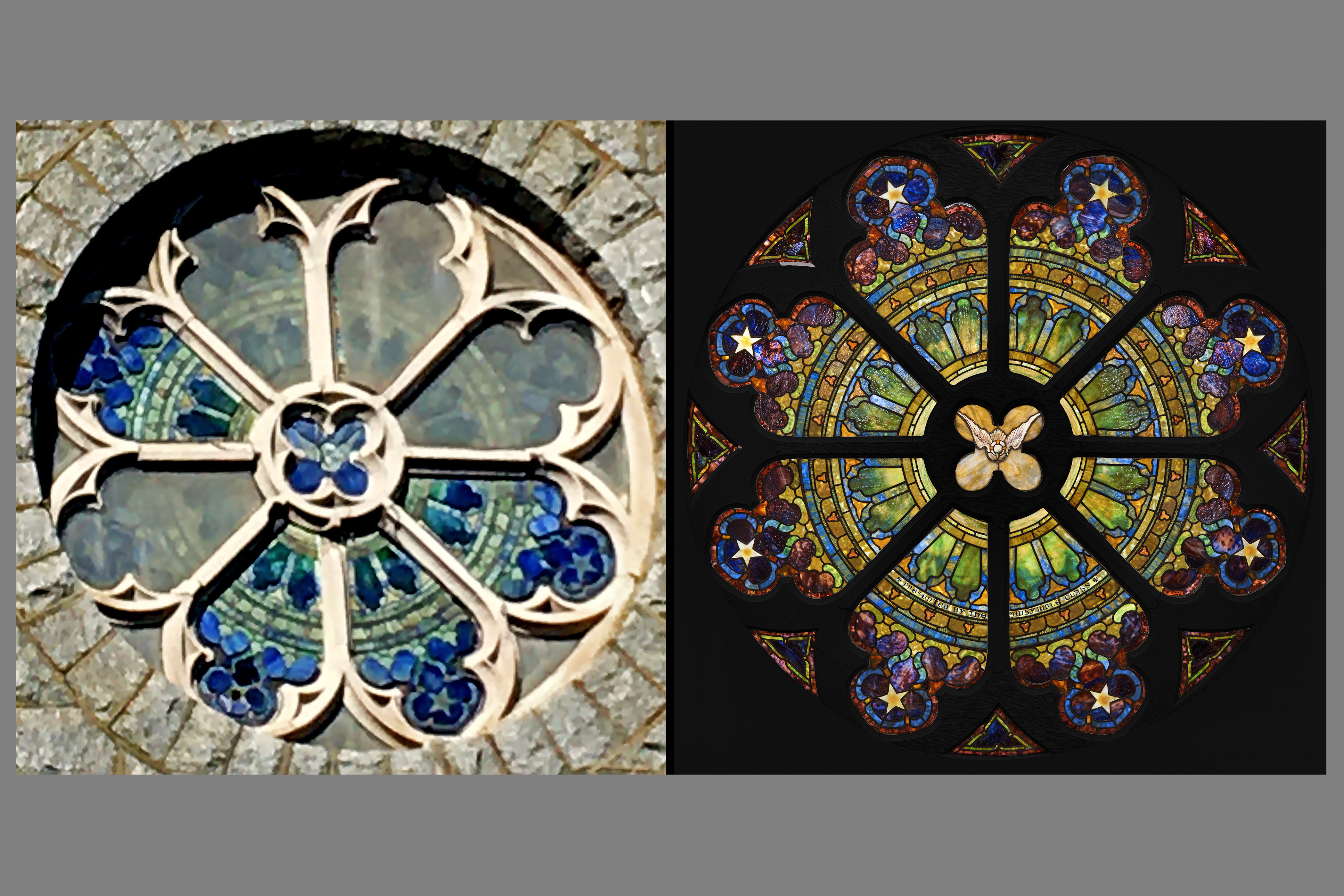The image showcases two beautiful, round stained glass windows set in a gray stone building. The window on the left appears to be viewed from the outside, partially obscured by dirt or light reflection, but you can still distinguish shades of blue and green emanating from it. It is encased in a circular stone frame, giving it a structured, yet artistic look resembling flower petals with concrete rings.

The right window presents a more vivid and detailed view from the inside, highlighting the full spectrum of stained glass colors including purple, green, blue, and yellow against a black background. Thick lines run diagonally, horizontally, and vertically, forming an intricate design that includes what appears to be a central butterfly motif with purple protruding arms and surrounding triangular patterns. Together, these side-by-side images contrast the subdued external view with the vibrant, ornate internal perspective, offering a comprehensive showcase of the windows' intricate artistry and colored illumination.